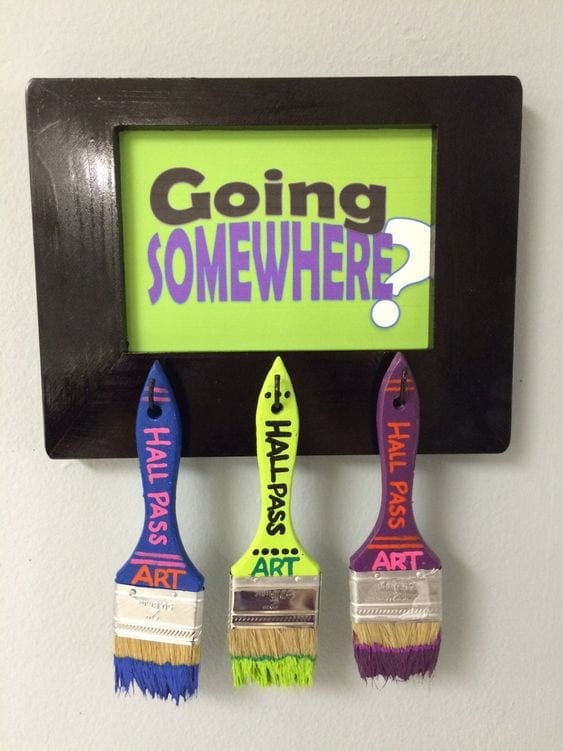The photograph showcases a charming and colorful setup likely designed for an art classroom. At the center is a bright green plaque framed in black, adorned with the question "Going somewhere?" The word "going" is in black, "somewhere" is in purple, and the question mark is white. Below this sign, three paintbrushes dangle from metal pegs, serving as creative hall passes. Each brush is not only vibrantly colored but also dipped in corresponding paints at the bristles: a blue brush with blue bristles and pink and orange writing, a lime green brush with green bristles, and a purple brush with purple bristles and red and pink writing. These brushes are labeled with "Hall Pass Art," making them easily recognizable and practical for students to use, while also being visually striking and unlikely to get lost. The entire setup is a testament to the teacher's ingenuity in repurposing old paintbrushes into functional and aesthetically pleasing tools for classroom management.